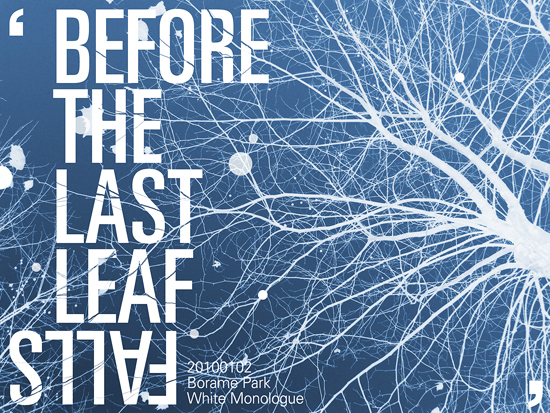The poster features a striking illustration against a dark sky blue background. On the right side, an intricate tangle of white tree branches sprawls in all directions, resembling a delicate, leafless network, with denser clusters near the center thinning out as they extend. The left side of the poster showcases text in prominent white font: "Before the last leaf falls," with the word "falls" notably written upside down. At the bottom center of the image, additional details are provided in a smaller font, indicating "20100102 Borem Park White Monologue."